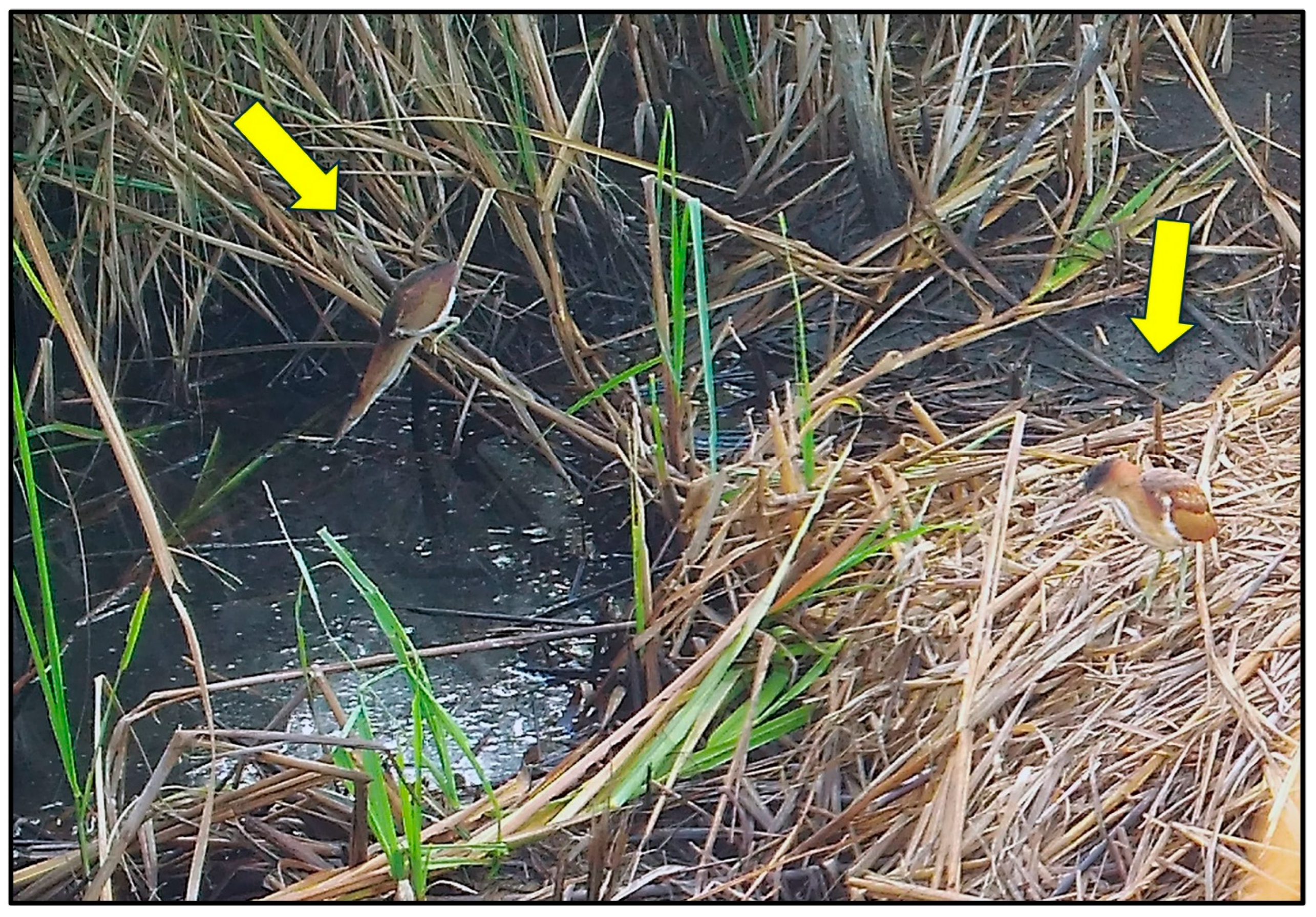The photograph captures a tranquil scene in a marsh or creek area, characterized by murky, greenish water surrounded by a mix of green and predominantly brown, dry grass or reed stalks. The water shows slight movement, indicating it's not entirely still. On the left side of the image, a yellow arrow points out a bird perched just above the water on a brown stalk. This bird features prominent long, skinny legs, a dark patch on its forehead, and blends into the environment with its brownish plumage. A second yellow arrow on the right side of the image highlights another bird closer to the camera standing amongst the reeds or hay-like grass. This bird also has spindly legs, and its feathers exhibit a mix of white and various shades of brown. The arrows are likely included to assist viewers in spotting both birds amidst the dense and varied vegetation.